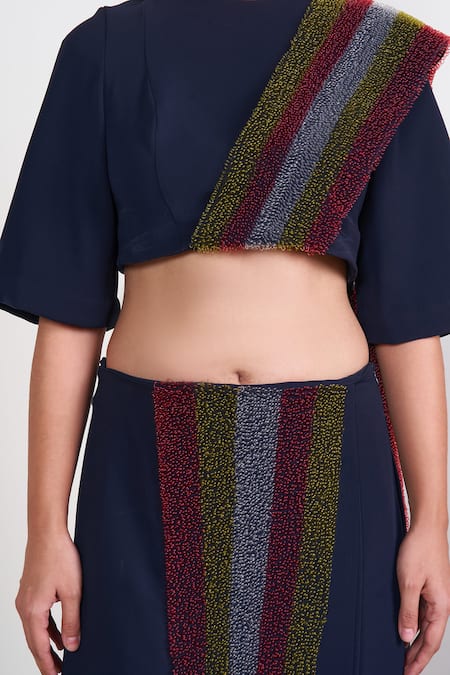The image portrays a person, likely a woman, modeling a distinctive outfit. The photo captures her from just below the neck to above the knees, highlighting a blue crop top that leaves her stomach exposed. The top has sleeves that extend down to her elbows, leaving her forearms visible. She's also wearing a blue skirt with a unique pattern.

A prominent feature of the attire is a sash, adorned with a vibrant array of stripes in green, maroon, blue, and once more green and maroon. The sash extends diagonally across her torso from one shoulder, crosses the exposed midriff, and is secured below the belly button, continuing the striping pattern onto the skirt area. The striped pattern is repeated down the middle of the skirt's crotch area, adding a coherent design element to the outfit. Overall, the combination of the blue fabric and colorful stripes gives the attire an eye-catching, multi-textured appearance.